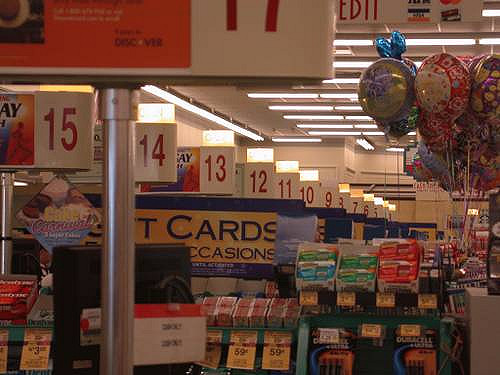This color photograph depicts the interior of a warmly lit grocery store. At the forefront, various shelves are stocked with items like candy, gum, and Duracell batteries. The aisle markers, white with red numbers, start at 15 and decrease sequentially down to 5, with aisles 3 and beyond visible in the distance. On the right side, a vibrant display of decorative party balloons adds a festive touch. The ceiling features long, white fluorescent lights, providing a steady glow. The store's walls are painted a yellowish shade, enhancing the warm atmosphere. Additionally, there are sections of merchandise dedicated to fruits, snacks, and gift cards, though no people or plants are visible in the scene.